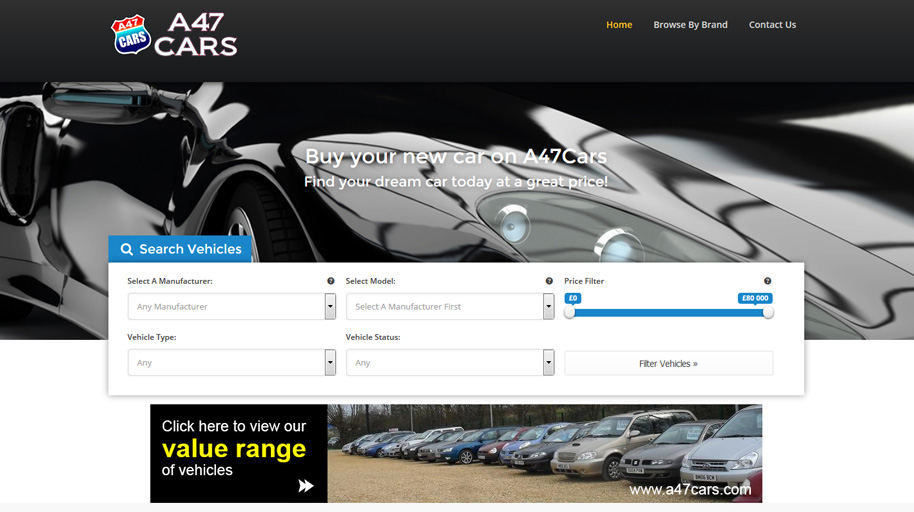The webpage for A47 Cars features a striking design that instantly captures attention. In the upper-left corner, there's a distinctive logo resembling a sheriff's badge or a Route 66 highway sign, divided into red and blue sections, with "A47 Cars" embossed in white text. To its right, "A47 Cars" is prominently displayed in bold letters.

Dominating the background is an image of a sleek, black sports car, radiating sophistication and power. Overlaying this backdrop is an inviting prompt: "Buy your car on A47 Cars. Find your dream car today at a great price." Beneath this call to action, a blue rectangle button labeled "Search Vehicles" beckons users to begin their search. The search interface includes drop-down menus for selecting a manufacturer and model, alongside a price filter featuring a blue sliding gauge ranging from £0 to £80,000. Additional categories for refining the search—like vehicle type and vehicle status—culminate in a "Filter Vehicles" button.

Below these search tools, a banner ad draws the eye with a black square on the left stating, "Click here to view our value range of vehicles." The words "value range" are emphasized in larger, yellow font. On the right, a panoramic display showcases a diverse array of cars—at least eleven—spanning a spectrum of colors from vibrant reds and blues to sophisticated blacks and golds. Lastly, the website address, www.a47.cars.com, is clearly displayed in the bottom left corner.